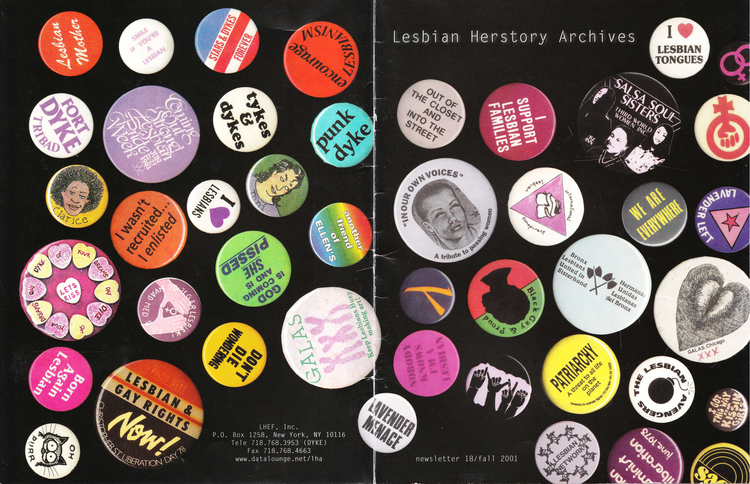The image depicts a collection of LGBTQ-themed buttons prominently displayed against a black background, showcasing their vibrant array of colors including turquoise, red, rainbow stripes, pink, neon green, white, yellow, orange, purple, red-and-green, and other assorted hues. Affixed to a poster, many of the buttons carry feminist or lesbian slogans and imagery. Notable examples include messages such as "I wasn't recruited, I enlisted," "I support lesbian families," "I ♥ Lesbian Tongues," and "Out of the closet and into the street." At the top right of the poster, the prominent text reads "Lesbian Herstory Archives," highlighting the focus on LGBTQ history and advocacy. Additionally, some text found near the bottom left of the image states "Newsletter 18 - Fall 2001," indicating a possible publication date and context for the display. The poster appears to have been folded, showing a visible crease in the middle.